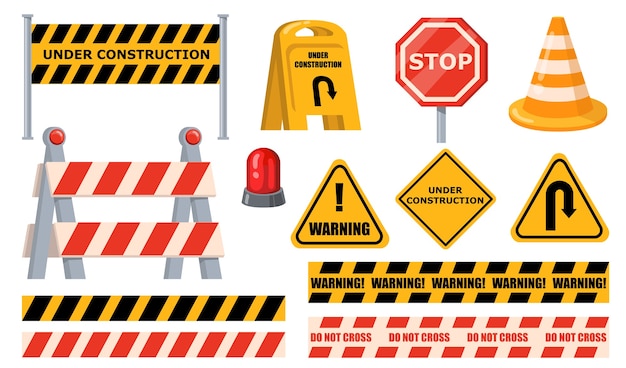This image is a detailed clip art sample featuring various types of construction and warning signs. In the top row, there are four items: a rectangular yellow and black "Under Construction" sign with black diagonal stripes, mounted on two silver poles; a yellow floor tent-style "Under Construction" sign with a U-turn arrow; a red octagonal stop sign; and an orange safety cone with three white stripes. The second row includes a construction sawhorse with red and white diagonal stripes and red reflectors, a red siren light on a gray base, a triangular yellow warning sign with an exclamation mark, a yellow diamond-shaped "Under Construction" sign, and another triangular yellow sign with a U-turn arrow. At the bottom are four stripes: a black and yellow striped rectangle, a red and white striped rectangle, a yellow and black one that repeats the word "Warning," and a red and white one that repeats the phrase "Do Not Cross." The arrangement and design provide a comprehensive representation of various signs typically used in construction zones.